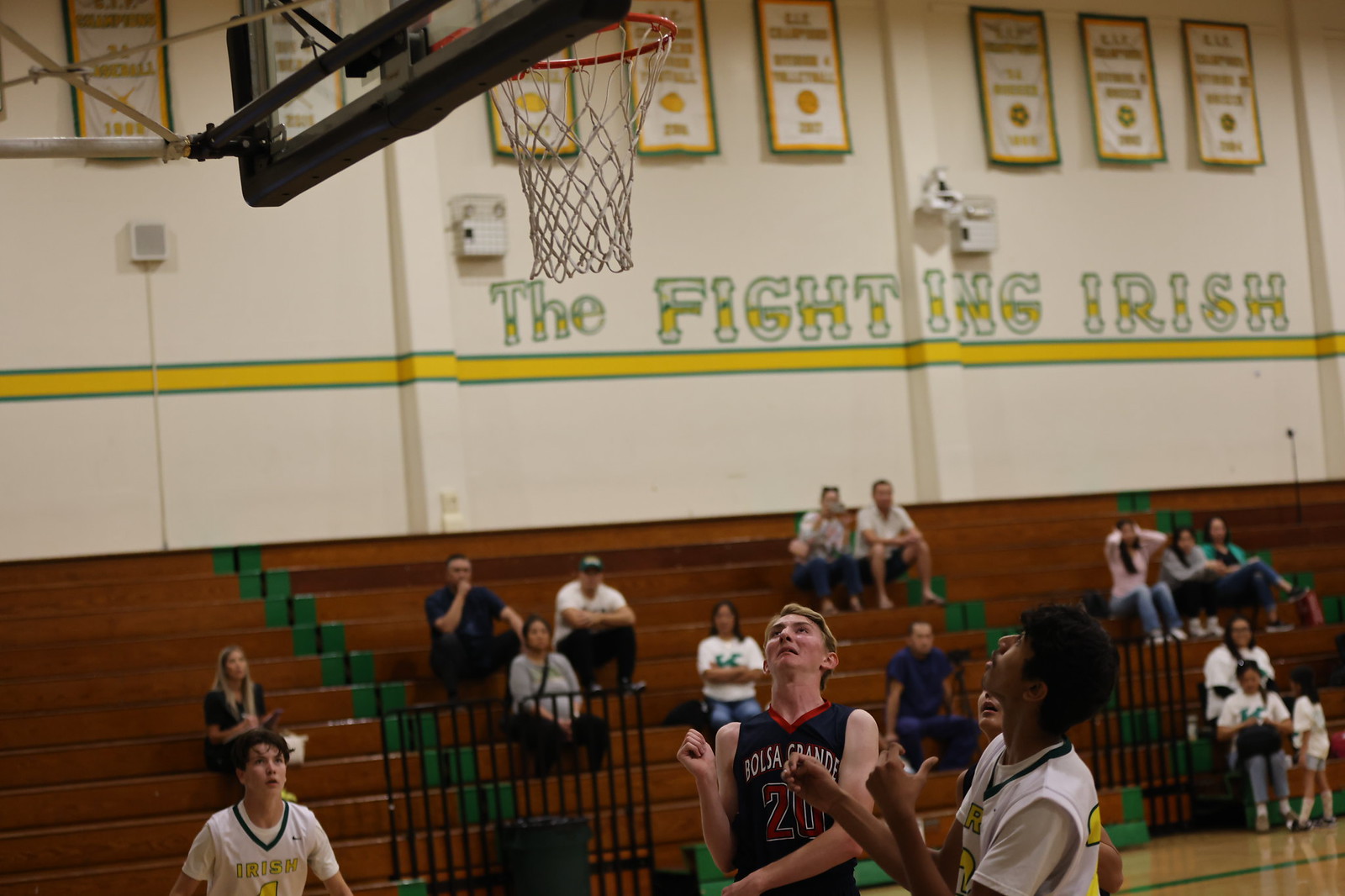The image captures an intense moment during a high school basketball game in a well-lit gymnasium. In the foreground, a group of boys are focused on the basketball hoop, though no ball is visible. A player in a dark navy jersey with white lettering and red numbers stands out as he is surrounded by teammates in white jerseys that have "Irish" written in yellow lettering outlined in green. The gym's wall prominently displays the words "Fighting Irish," underlined by a yellow stripe with green outlines. Above the phrase are posters listing years and championships, contributing to the competitive atmosphere. Spectators can be seen sitting in the stands, adding to the vibrant scene. The basketball hoop is positioned on the upper left side of the image.